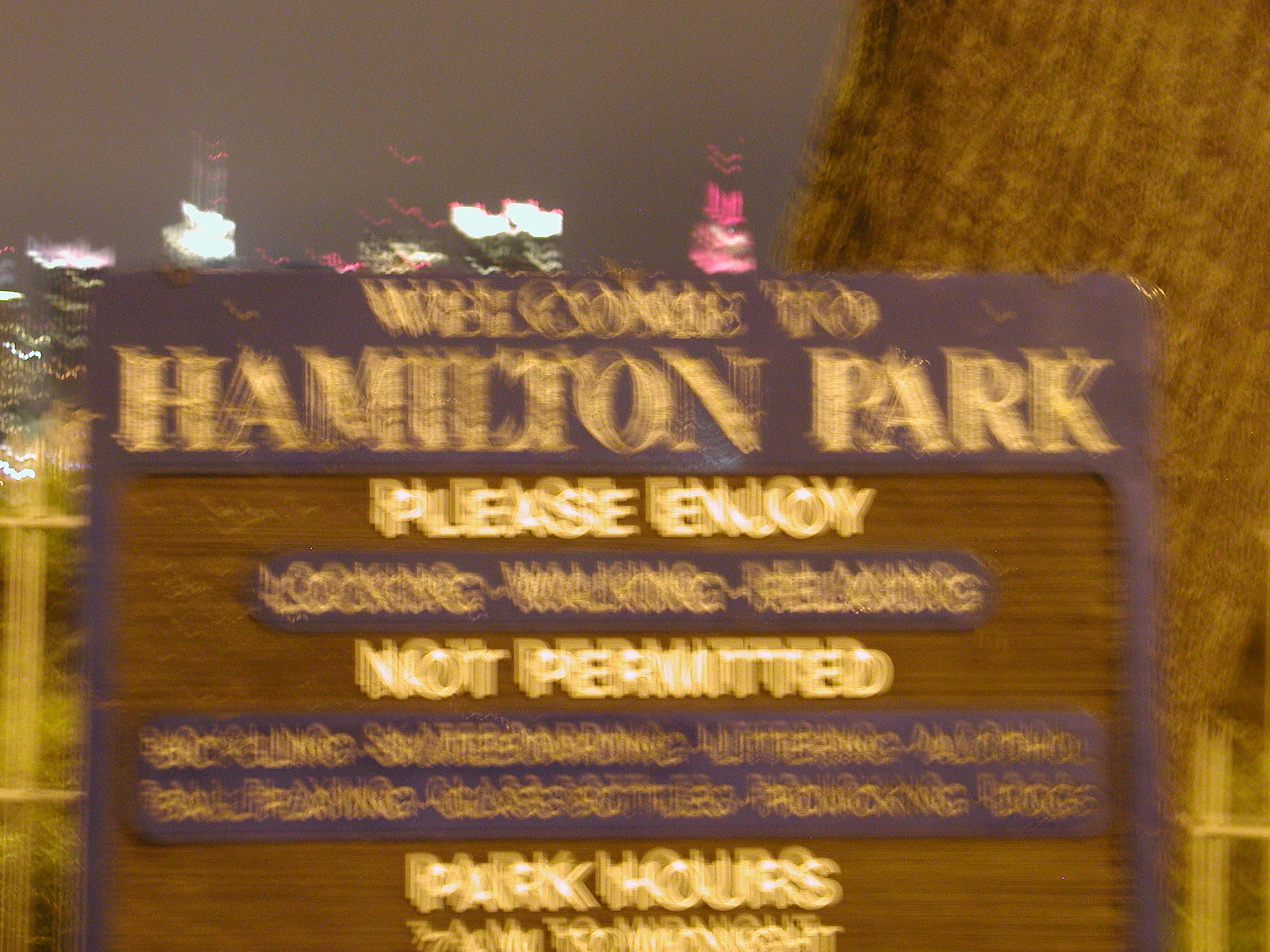The outdoor nighttime photograph is heavily blurred and grainy, making details challenging to decipher. The focal point of the image is a wooden sign with gold lettering that reads "Welcome to Hamilton Park" at the top. Below, a rectangular inlay features yellow lettering with the partially readable message, "Please enjoy looking, walking, relaxing," followed by an unreadable segment and the words "not permitted." Further down, it mentions "park hours," but the specifics are indiscernible due to the blur. The sign is framed in dark brown, and there are white and pink flowers visible above and around it. In the background, the upper left shows a cityscape with illuminated skyscrapers topped with communication antennas. To the right of center, a large tree with a multi-toned trunk extends from behind the sign, exiting the frame at the upper right corner. The image suggests the camera was moving, contributing to the significant blur and graininess.